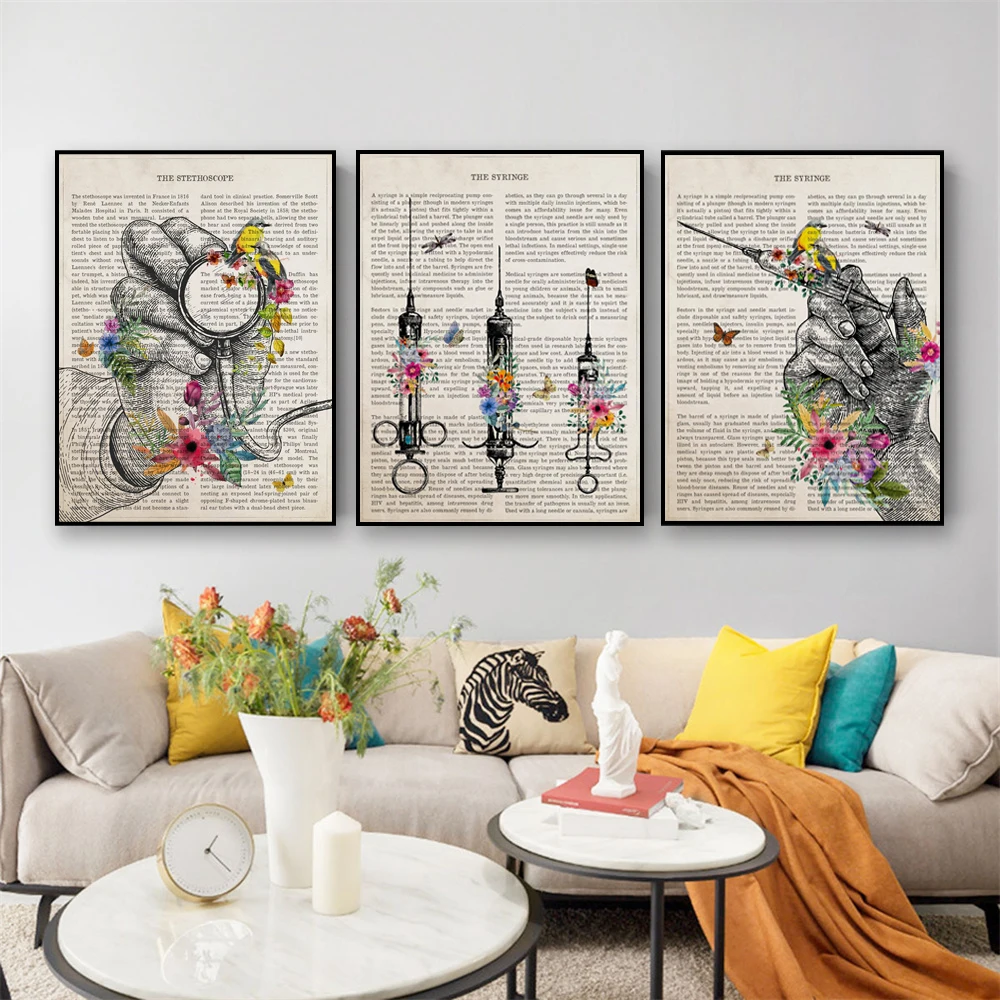The photograph captures a cozy family room dominated by three artistically framed pictures on a white wall, each illustrating different medical themes. The left picture, titled "The Stethoscope," features a hand holding a stethoscope surrounded by colorful flowers and a yellow bird with a blue head. The middle picture highlights three old-fashioned syringes from the 18th and 19th centuries, adorned with flowers. The right picture depicts a hand holding a syringe, accompanied by birds, butterflies, and flowers, echoing the artistic, medical motif.

Below these frames is a comfortable couch embellished with various pillows, including a distinctive one with a zebra head design. An orange blanket or cover is draped partially over the sofa and onto the gray carpet. The room's decor includes two circular black tables with marble-like surfaces. One table holds a stack of books topped with a miniature Greek-style statue, while the other hosts a carriage clock and a potted plant. The scene is warmly lit, emphasizing the room's blend of artistic and homely elements.